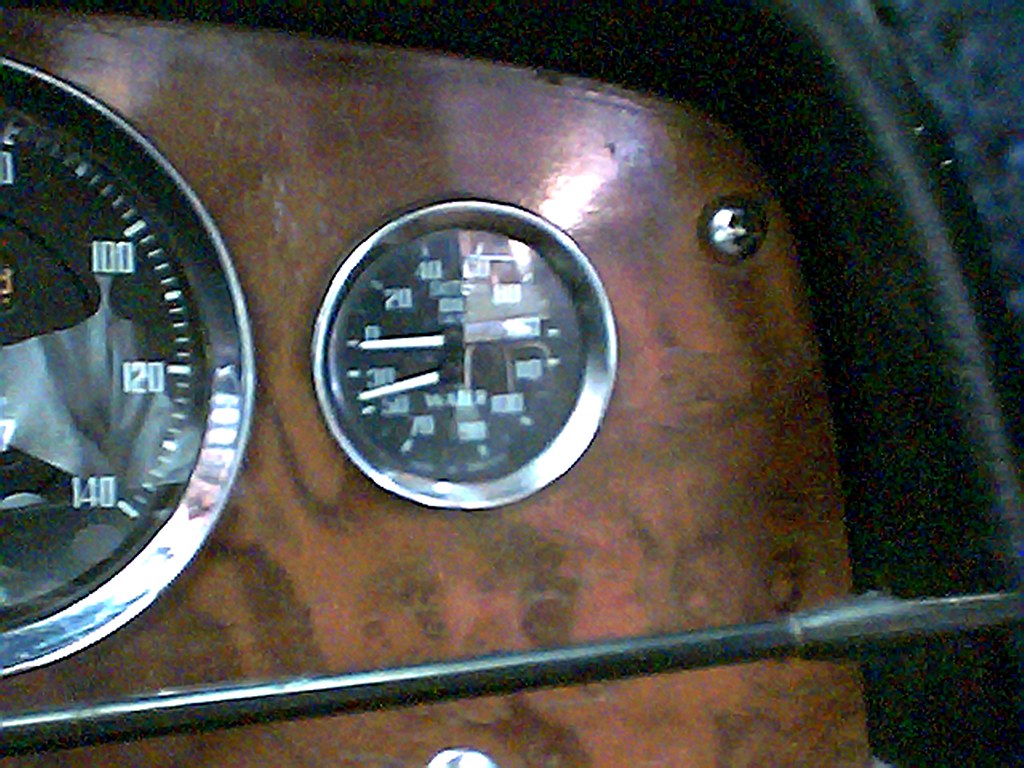The close-up image captures a somewhat grainy view of a car's dashboard, slightly distorted due to poor image quality. The dashboard is framed by a dark black vinyl border, exhibiting an artifacting pattern of green, yellow, blue, and red dots, likely caused by the camera's ISO settings. A slender, silver metal rod extends towards the right, presumably connected to the steering wheel. The dashboard features a reddish-brown wooden panel with a darker brown gradient, fastened in the upper right corner by a visible silver screw. Two silver-rimmed dials are present; the left one is a speedometer, marked with increments ending at 100, 120, and 140. The right dial is obscured by glare, making its markings difficult to discern, but it appears to display two sets of measurements, the lower needle ranging from 30 to 100, and the upper needle from 0 to 100.